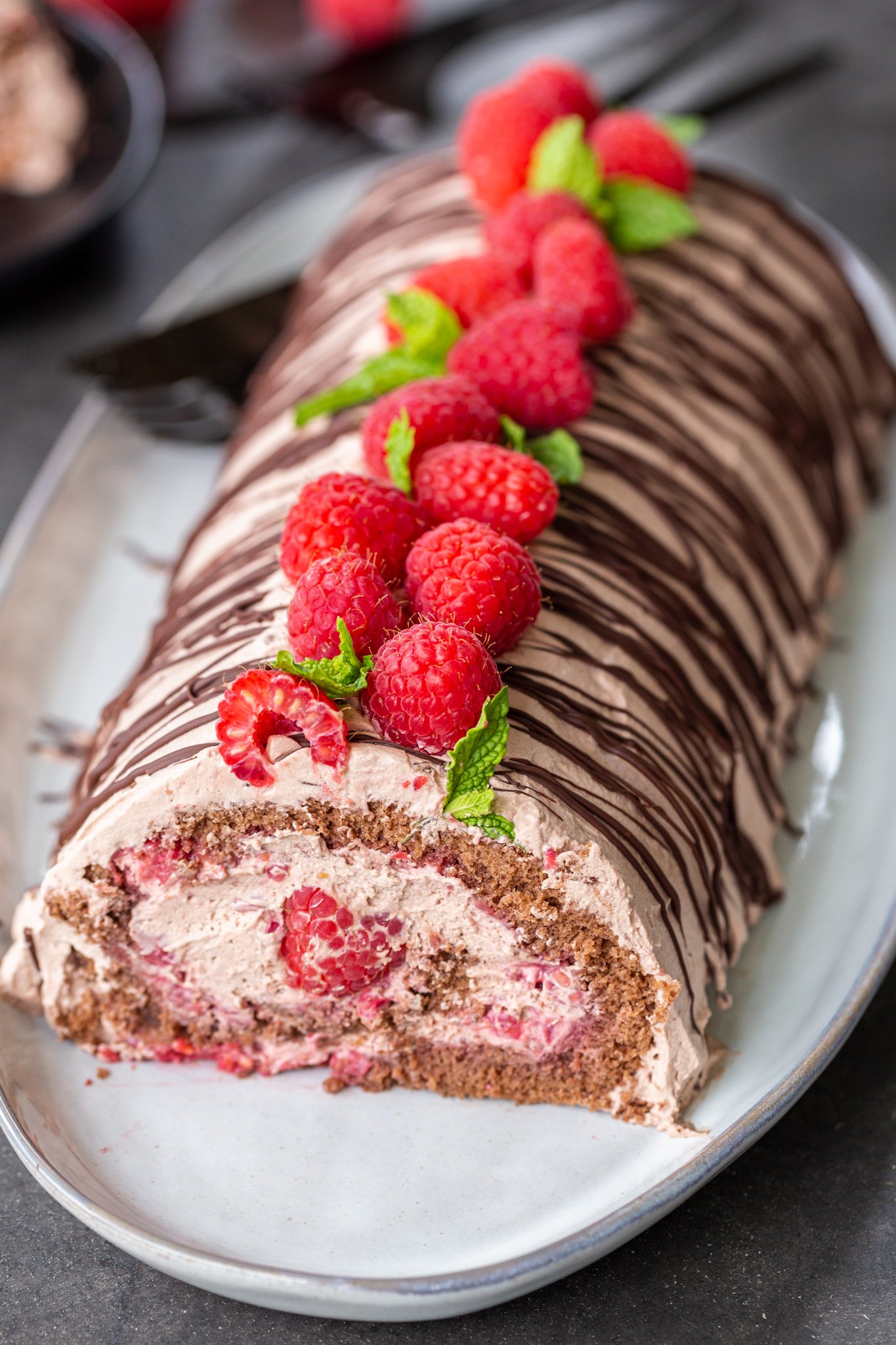This photograph showcases a beautifully presented dessert cake, positioned on a white oval plate against a dark, blurry background. The cake, resembling a rolled Yule log often associated with Christmas, is elegantly decorated with vibrant red raspberries and fresh neon green mint leaves. Its exterior is covered in light brown mousse with delicate chocolate drizzle artfully piped on top. The cake has been sliced open, revealing its intricate layers: a central core of bright raspberries, surrounded by a creamy pink mousse, encased within a light brown sponge cake, and another layer of mousse hugging the exterior. The foreground captures the dessert's compelling details, including a somewhat obscured black utensil at the end of the plate. The clear colors of white, red, and brown dominate the visual, making the dessert appear delightfully appetizing.